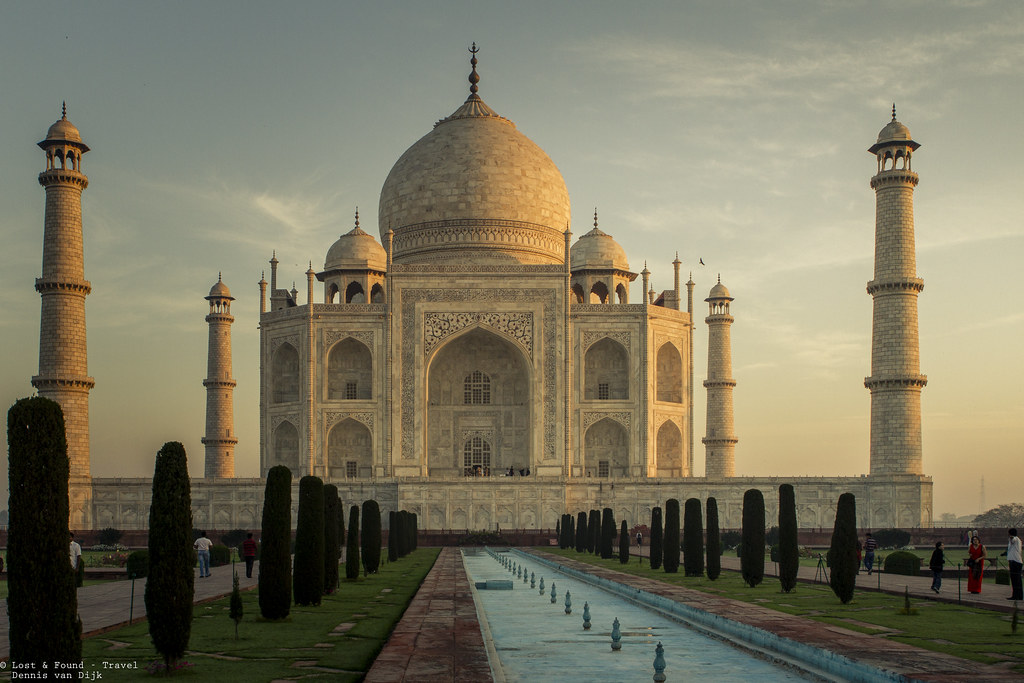This is a stunning wide shot of the Taj Mahal, captured around sunset, likely between 5 to 6 p.m. The majestic monument, an iconic white and light gray structure with light brown tints, stands prominently with its large central dome flanked by two smaller domes. There are also four minarets, each topped with smaller domes, located at the corners of the structure. The foreground features a long, pristine reflecting pool flanked by two rows of tall, cigar-shaped trees, leading the eye toward the grandeur of the Taj Mahal. The lawn is a deep green, meticulously maintained, with red brick walkways for pedestrians on either side of the pool. Scattered around are people, some capturing photos and others approaching the monument. The background includes a small tower and some greenery, contributing to the serene setting. The sky exhibits hues of light blue and gray, tinged with amber from the setting sun, casting a warm glow on the Taj Mahal and enhancing its ethereal beauty.